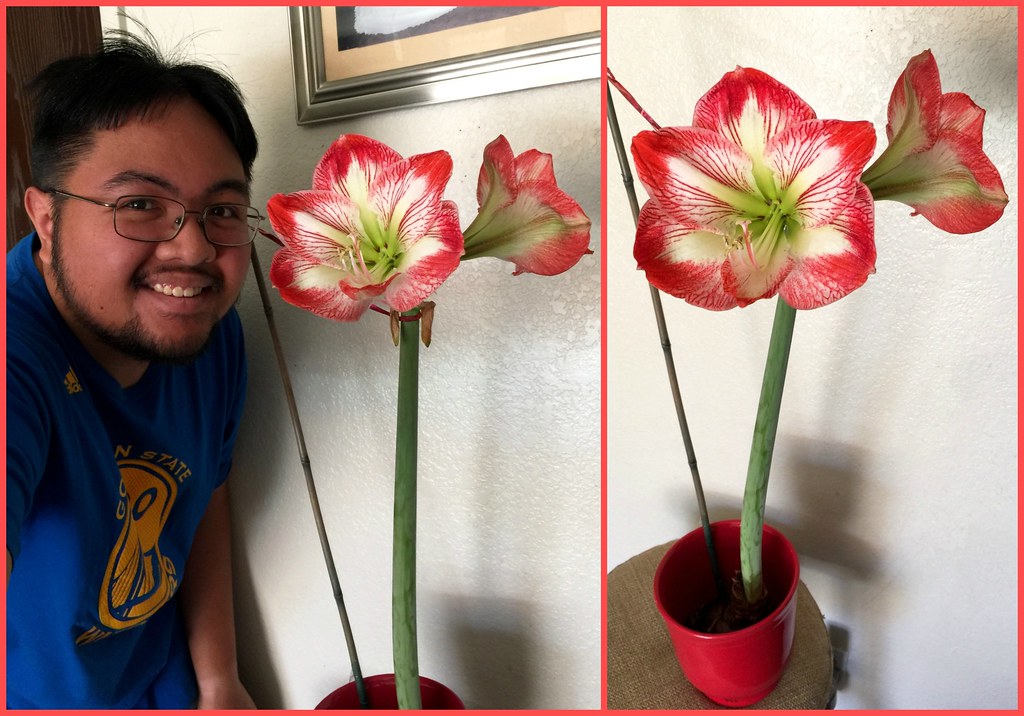The larger image on the left showcases a young bearded man with short black hair and black wire-rimmed glasses, smiling proudly at the camera next to a blooming amaryllis plant. He is wearing a blue Golden State Warriors t-shirt with yellow lettering. The amaryllis features striking red petals with white centers and is supported by a bamboo stake tied to its long green stem, planted in a glossy maroon or brick red ceramic pot. The scene is set against a textured white wall, with the bottom part of a framed and matted piece of artwork visible in the background. The smaller image on the right is a close-up of the amaryllis, focusing on its vibrant flowers and the supporting stake. The flower pot sits on a small brown tabletop, which is only visible in this tighter shot. This right-hand image captures the intricate details of the amaryllis flowers, highlighting one flower facing the camera and another angled away, emphasizing the plant's striking contrast of colors.